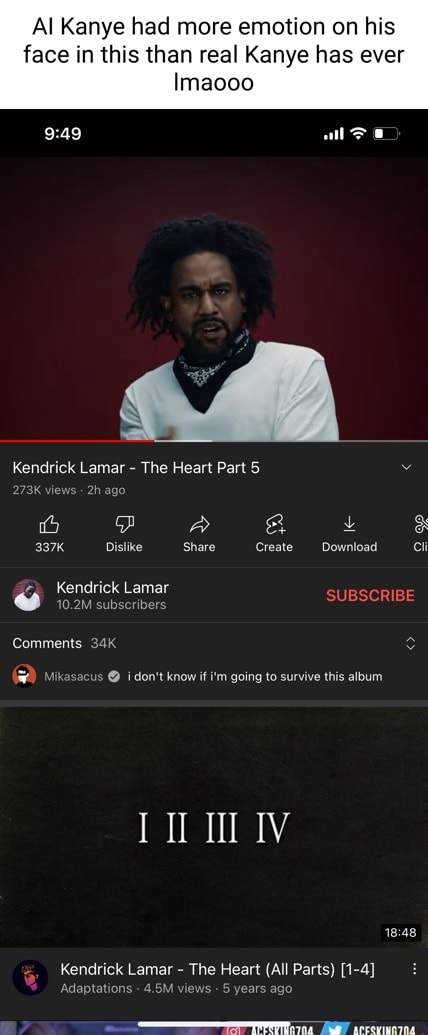This image is a screenshot of a cell phone displaying Kendrick Lamar's YouTube channel. The screen features a video titled "The Heart Part 5," which has garnered 273,000 views and 337 likes within just two hours of being posted. The video duration is 18 minutes and 48 seconds. Below the video, various interactive buttons are visible, including options to dislike, share, create, and download the video.

Kendrick Lamar's channel name is prominently displayed, boasting an impressive 10.2 million subscribers. The profile picture next to the channel name shows Kendrick Lamar wearing a white t-shirt. Also visible is a subscribe button to the right of his profile picture. Scrolling further down, there's a highlighted user comment stating, "I don't know if I'm going to survive this album."